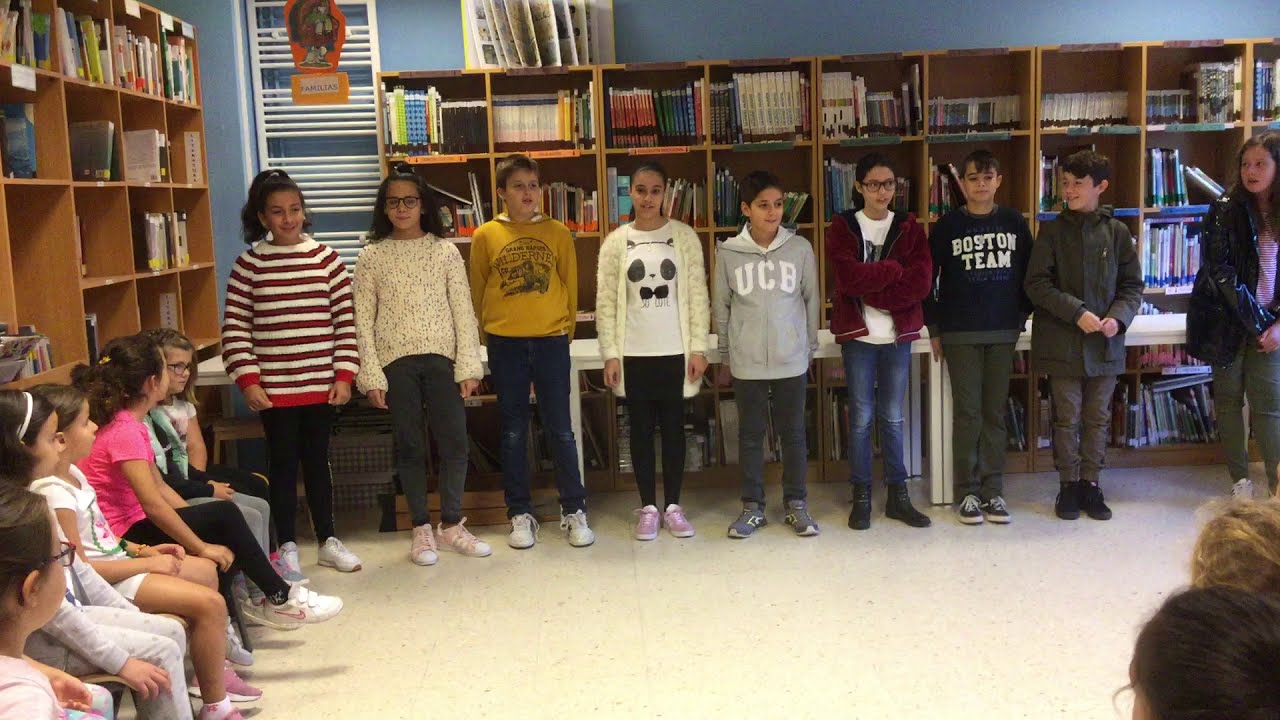This indoor photograph captures a diverse group of school children, likely around 10 years old, standing in a horizontal line in what appears to be a school library or a similar resource room. The backdrop of the image consists of walls lined with shelves, mostly filled with books but also interspersed with binders and games. The wall behind the shelves is a grayish-blue color.

In the foreground, from left to right, the children are dressed in various attire. The first child, an African or Hispanic girl, is wearing a red and white vertically striped long-sleeve sweater over black leggings. Next is a girl with dark hair pulled back, wearing dark-rimmed glasses, a white cable-knit sweater, and dark pants or leggings. Following her is a boy in a mustard gold sweatshirt with a graphic image, blue jeans, and white sneakers; he appears to be Caucasian with dark brown hair.

At the center of the row stands a girl in a white t-shirt with an indiscernible black and white graphic under a white cardigan sweater and black pants, also wearing white sneakers. To her right, a boy in a gray hoodie with "UCB" in white lettering and gray or black jeans stands, possibly of Hispanic or Middle Eastern descent. Next, a girl slightly taller than the previous boy, is wearing a maroon sweater over a white t-shirt, stonewashed blue jeans, and dark sneakers, with her dark hair pulled back and dark-rimmed glasses.

Continuing left to right, a boy with dark brown hair falling over his forehead, dressed in a black t-shirt with "Boston Teen" in white writing, black or dark gray pants, and gray sneakers, stands next to another Caucasian boy wearing a gray or olive drab jacket over gray jeans and black sneakers. This boy is looking slightly to his right. On the very far right of the image stands an indiscernible figure, possibly a teacher or moderator, who is farther back in the background.

In addition to the standing children, a row of similarly aged children is seated along the left side of the photograph, appearing to watch the standing children, possibly engaged in some form of recitation, reading, or presentation. The lower right corner reveals the heads of a couple more audience members. The entire scene suggests an organized performance or presentation within the school's library environment.